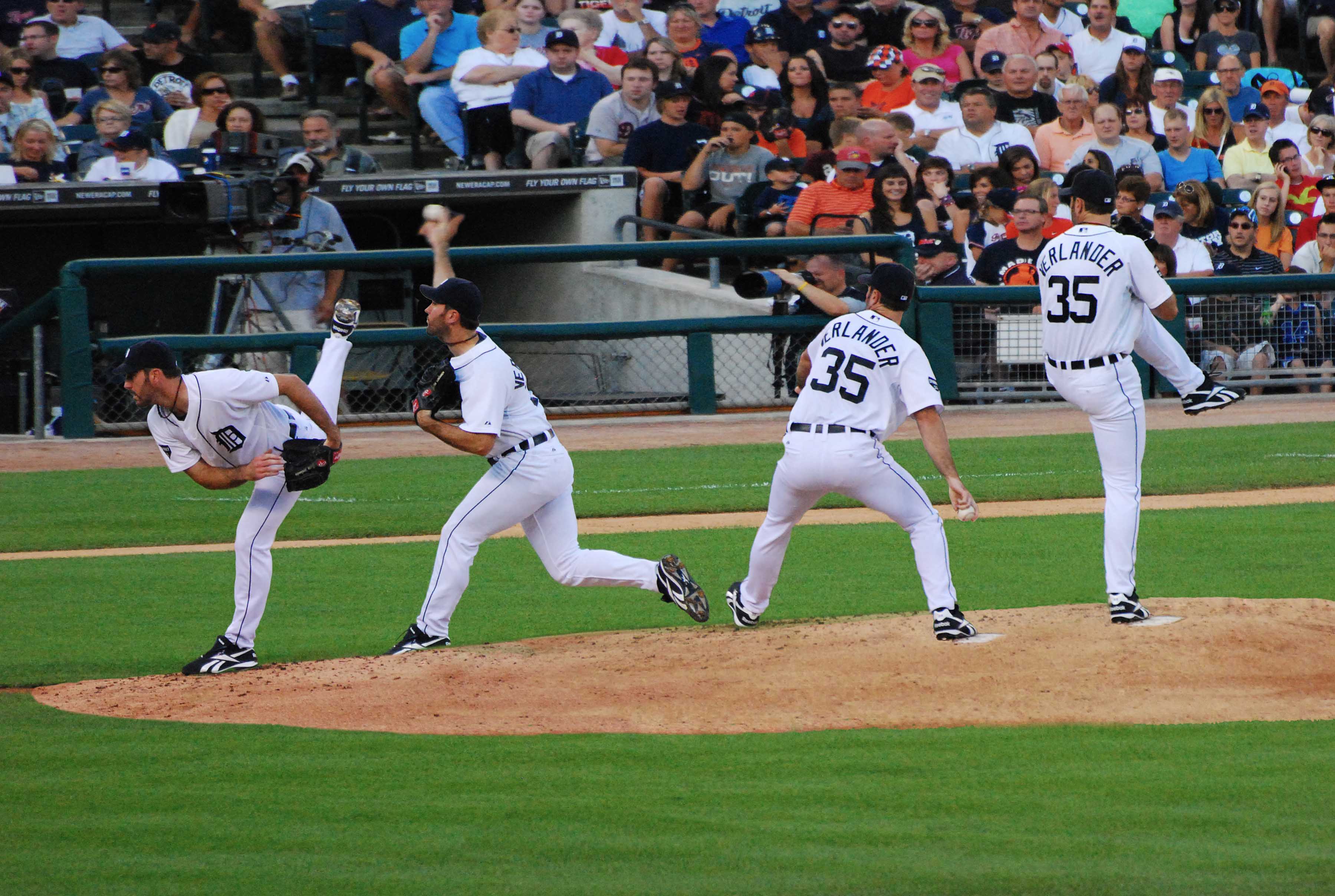The image is a detailed color photograph of baseball pitcher Justin Verlander during his tenure with the Detroit Tigers, showcasing a time-lapse sequence of his pitching motion. Though it creates an illusion of four distinct pitchers on the mound, it is indeed only one pitcher depicted in various stages of throwing a pitch. The series begins with Verlander winding up with his knee raised, proceeding to step forward, arm coming around, and culminating in the release of the pitch. Viewed from a side angle, likely from around first base, the photo captures the lush green grass of the field and the pitcher's mound. Verlander is clad in a white uniform featuring dark blue or black lettering and the number 35. The background reveals a bustling stadium with spectators in the stands, and a cameraman positioned in the dugout documenting the game. This photograph masterfully illustrates the fluid and dynamic movement of a major league pitcher in action.